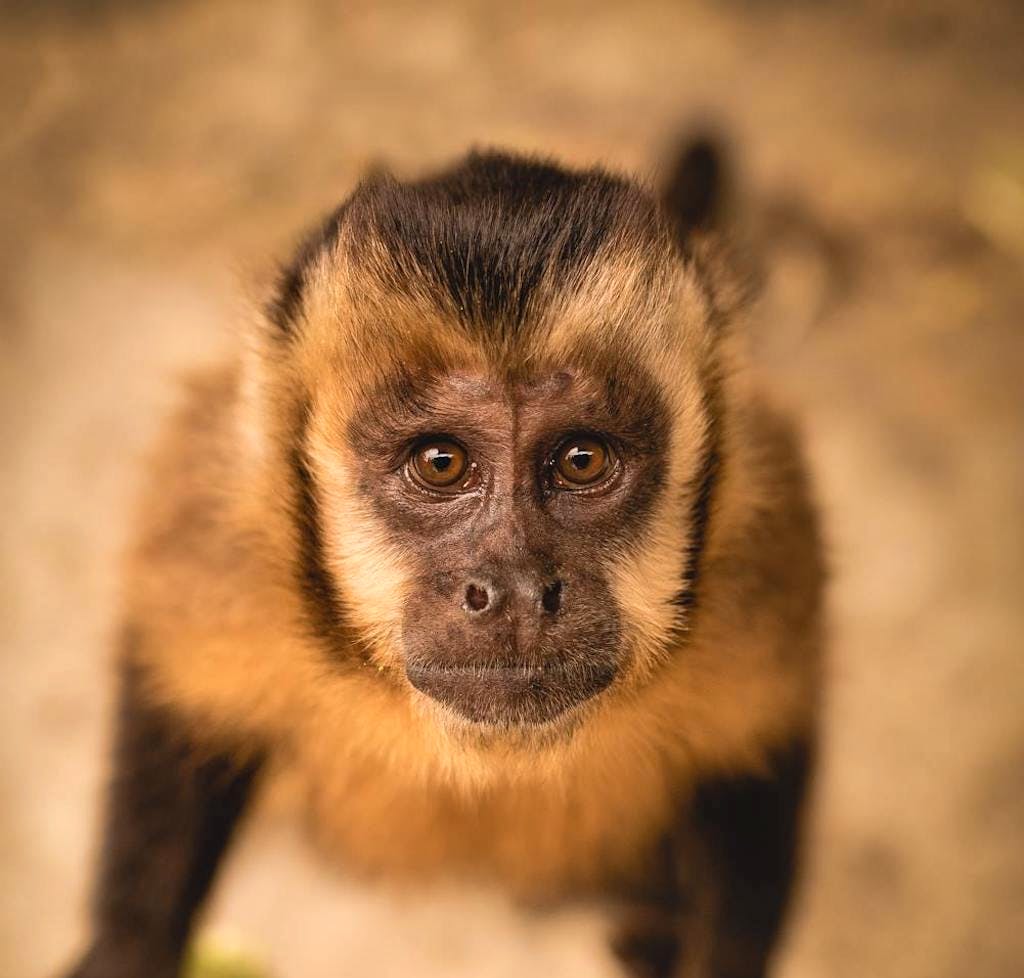This is a close-up image of a small monkey, likely a macaque. The monkey's face, the focal point of the image, is adorned with light brown fur and framed by slightly darker brown fur. The creature's large, round eyes, possibly hazel, stare directly into the camera, giving it an intent and inquisitive expression. The bridge of its nose is also covered in fur, while the nostrils are distinctly visible. Its mouth is closed, and you can see tiny, prominent hairs sprouting from its chin. The body of the monkey is out of focus, but discernible patterns in its fur can be noted: light-colored around the torso and darker on the arms, legs, and the end of the tail. The background of the image is a completely out-of-focus tan color, ensuring all attention remains on the monkey's expressive and detailed face.